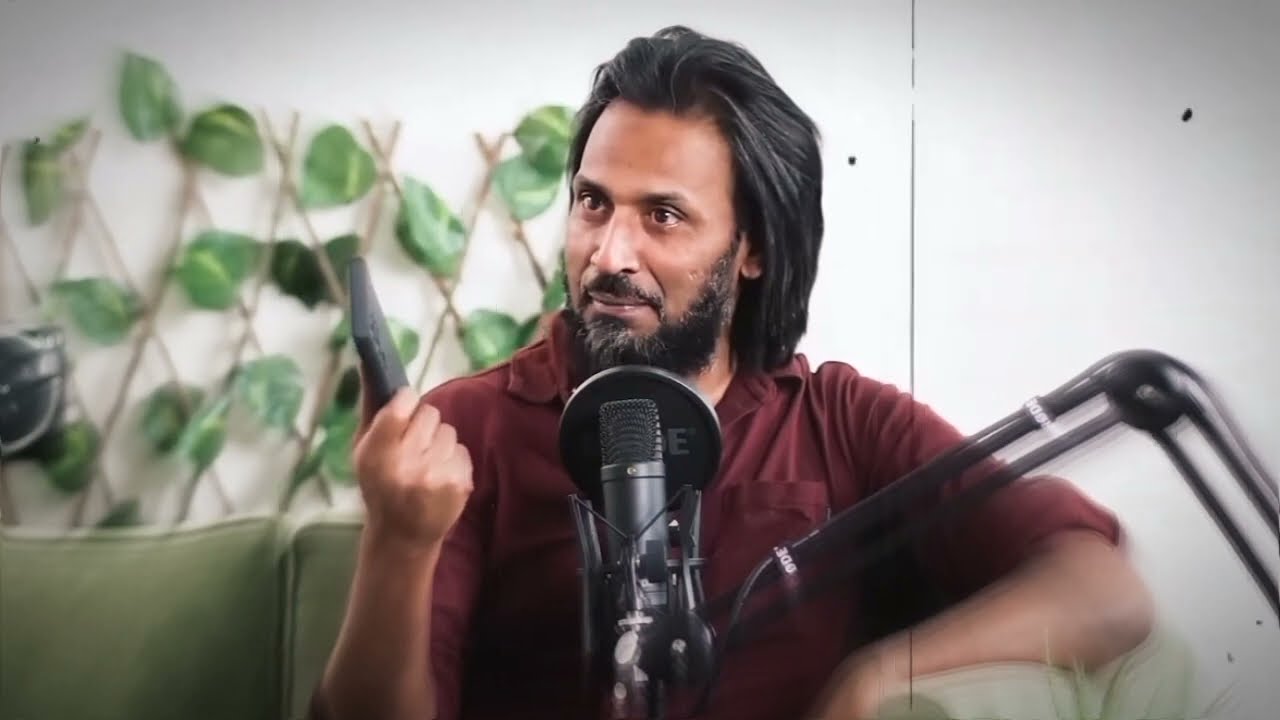The image captures a man seated indoors, likely in a recording studio or on a television set. He is talking into a large black microphone mounted on an extended arm that angles into the image from the side. The man has long black hair combed back, a dark beard flecked with gray, and tanned skin. He is wearing a maroon short-sleeved shirt with a collar and a pocket. His right hand clutches a dark-colored cell phone, and he appears to be looking at it curiously while engaged in conversation. He is seated on a pale green or beige couch, with the visible arm of the couch supporting his tanned left arm. Behind him, there is a white or off-white wall adorned with latticework featuring fake green leaves and brown twigs arranged in a diamond pattern, adding a decorative touch to the background.